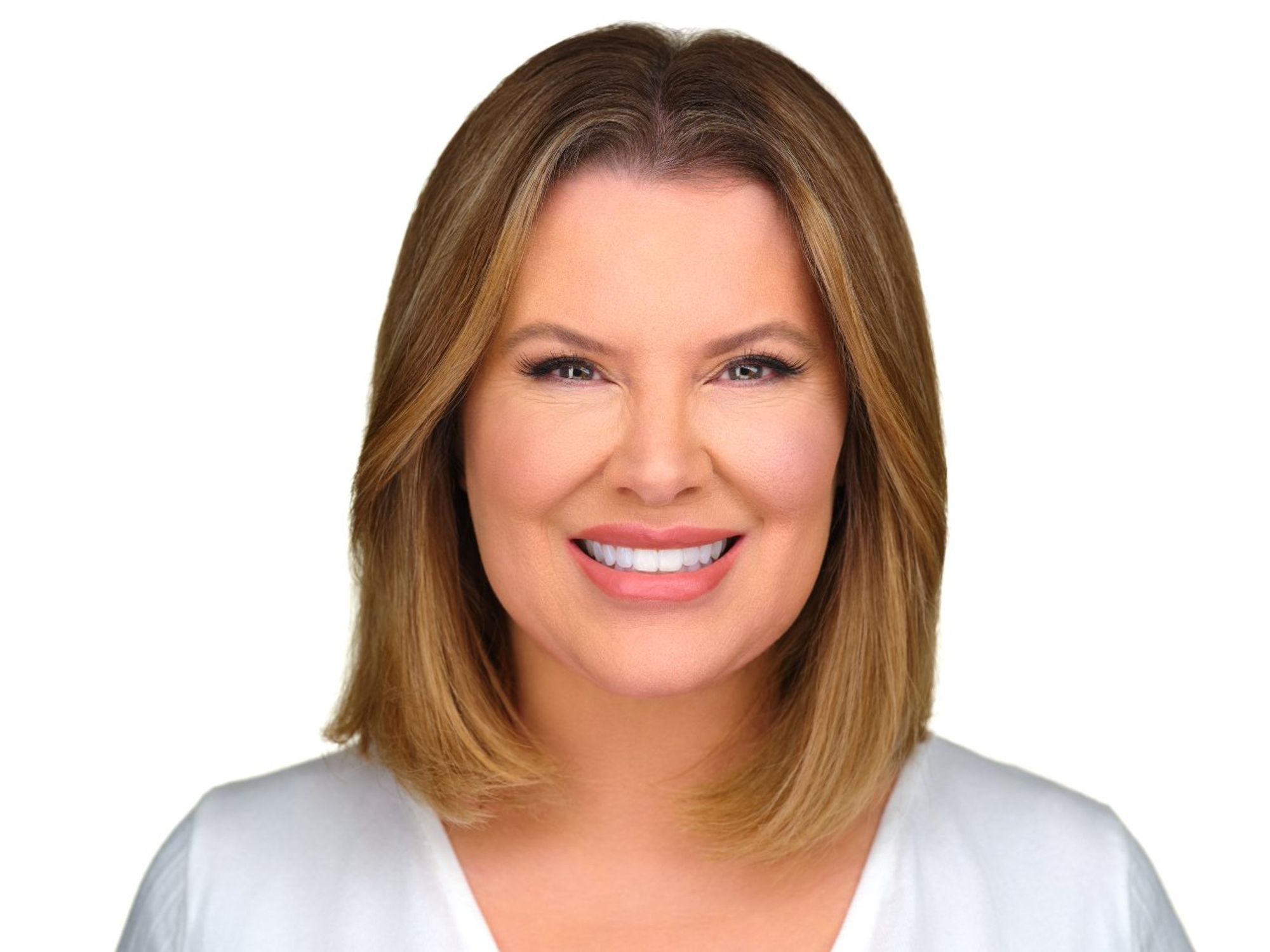This is a close-up headshot of an attractive middle-aged woman named Casey Curry, who is the Senior Director of Strategic Communications and Philanthropy. She radiates happiness with a bright, white smile that reveals her straight teeth and barely shows a part of the bottom row. Casey has very straight, shoulder-length honey blonde hair with golden highlights and some subtle traces of gray, parted neatly in the middle. Her fair complexion is complemented by a foundation makeup, and she wears a pale-pink lipstick that enhances her natural smile lines and crow's feet, suggesting she smiles often. Her expressive green eyes are framed by long lashes and well-arched eyebrows. Casey is dressed casually in a white v-neck shirt, adding to her approachable and professional appearance. The image is set against a simple white background, capturing her facing directly toward the camera in a large-scale, detailed photograph.